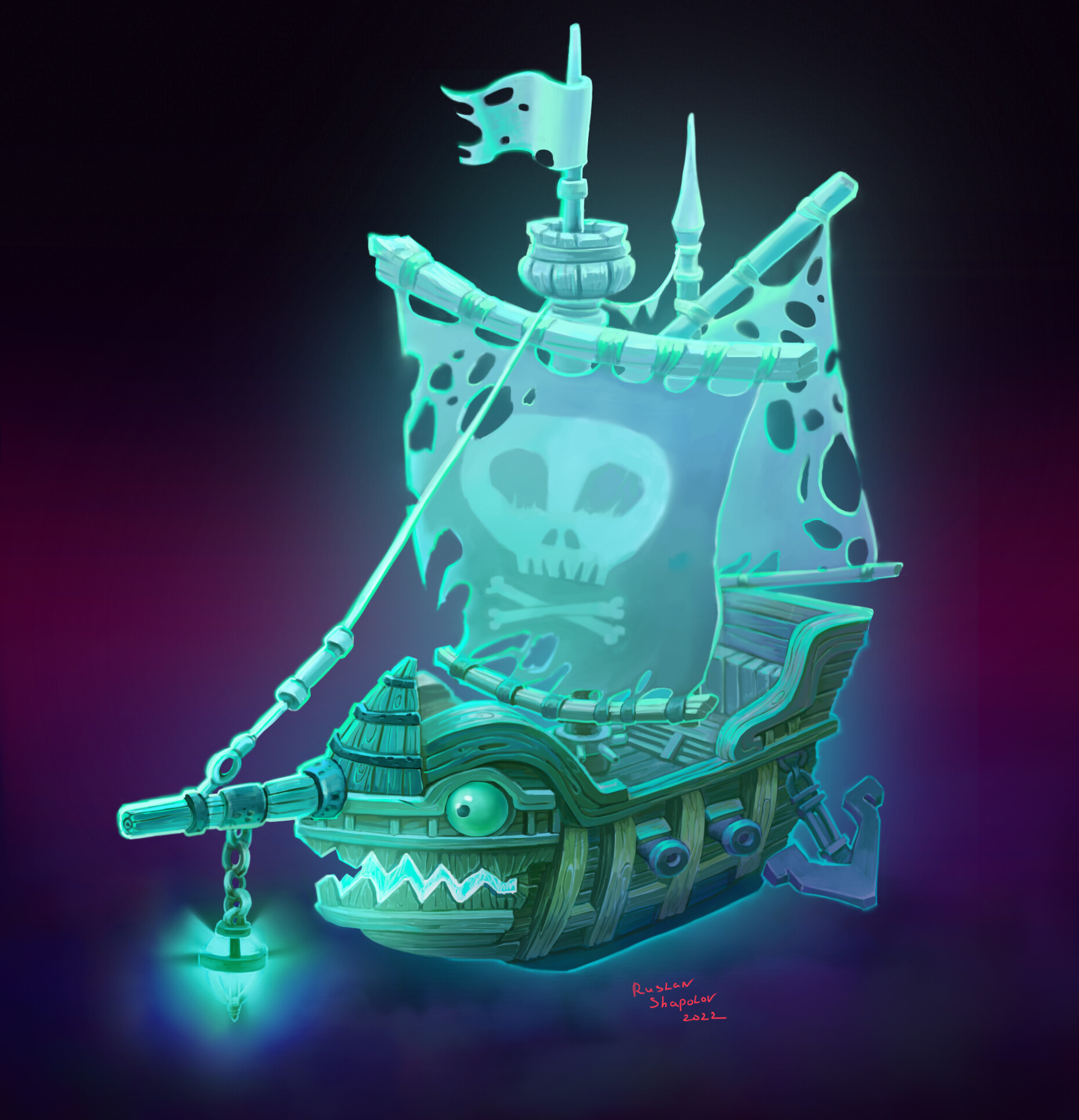The poster in front of me features a detailed, computer-generated image with a dark, purplish, and bluish background that transitions from black at the bottom, creating a gradient effect. Dominating the foreground is an animated, science fiction-inspired pirate ship, depicted with almost sentient characteristics. The ship's prow features menacing eyes and an evil grin, giving it an anthropomorphic appearance. Acting as a nose on the front is an extended section, from which an anchor dangles precariously.

The ship is primarily green and appears illuminated, with some red script or writing across the center lower section. Both sides of the ship fade into darkness, accented by a subtle red hue emanating from the right side of the image. The mast displays a tattered flag bearing the iconic skull and crossbones, signifying its pirate nature. Further back, another mast with a flagpole is visible, this second flag also worn and full of holes, suggesting a history of tumultuous weather and battles. The ship's overall condition, with its shredded and weathered sails, indicates it has endured many hardships on its voyages.